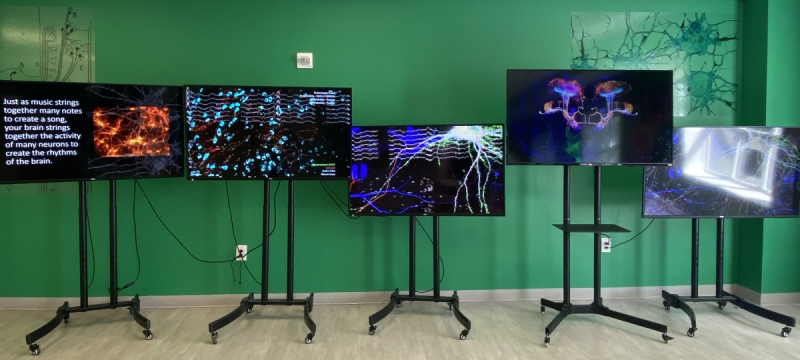This color photograph captures a setup of five computer monitors on rolling stands arranged beside each other against a green wall. Each monitor displays a different visual, and some stands are taller while others are shorter. The far-left monitor shows text that reads, "Just as music strings together many notes to create a song, your brain strings together the activity of many neurons to create the rhythms of the brain," accompanied by a bright orange and yellow pattern. The next monitor features many blue dots with unreadable writing. The third monitor displays a white, lightning-like pattern with blue and wavy lines. The fourth monitor shows a computer-animated mushroom-like object, while the final monitor depicts a brightly lit photograph of a window. Each monitor is plugged into electrical outlets near the wall's base, with visible cords and wires. The room, simple in design, also features a couple of paintings or pictures on the wall. There are no people present in the photograph.